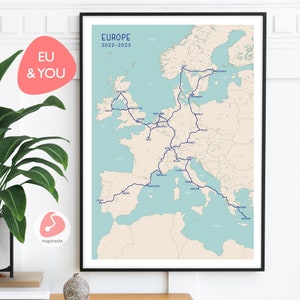The image depicts a framed map of Europe for the years 2022 to 2023, prominently displaying the title in blue text at the top left. The map itself features teal-colored waters and cream-colored land masses. Across the map, blue lines — likely representing train routes or connections — link various countries, extending even over large bodies of water. The map is encased in a frame with a white border and a black outer edge, set against a white brick wall.

In the top left corner, there is an oblong pink shape resembling a guitar pick, marked with the text "EU and you" in blue. At the bottom left, there is another pink guitar pick-shaped figure along with a white circle. Below these shapes, a white squiggly line with a ball at the end is present, accompanied by some black text that is unreadable due to its blurriness.

Additionally, there appears to be more context around the map: a plant with a white pot featuring green leaves sits on a nearby counter or shelf. Below the map, another shelf is visible, seemingly holding an object that might be a rock or another item that potentially lights up, although this detail is less clear.